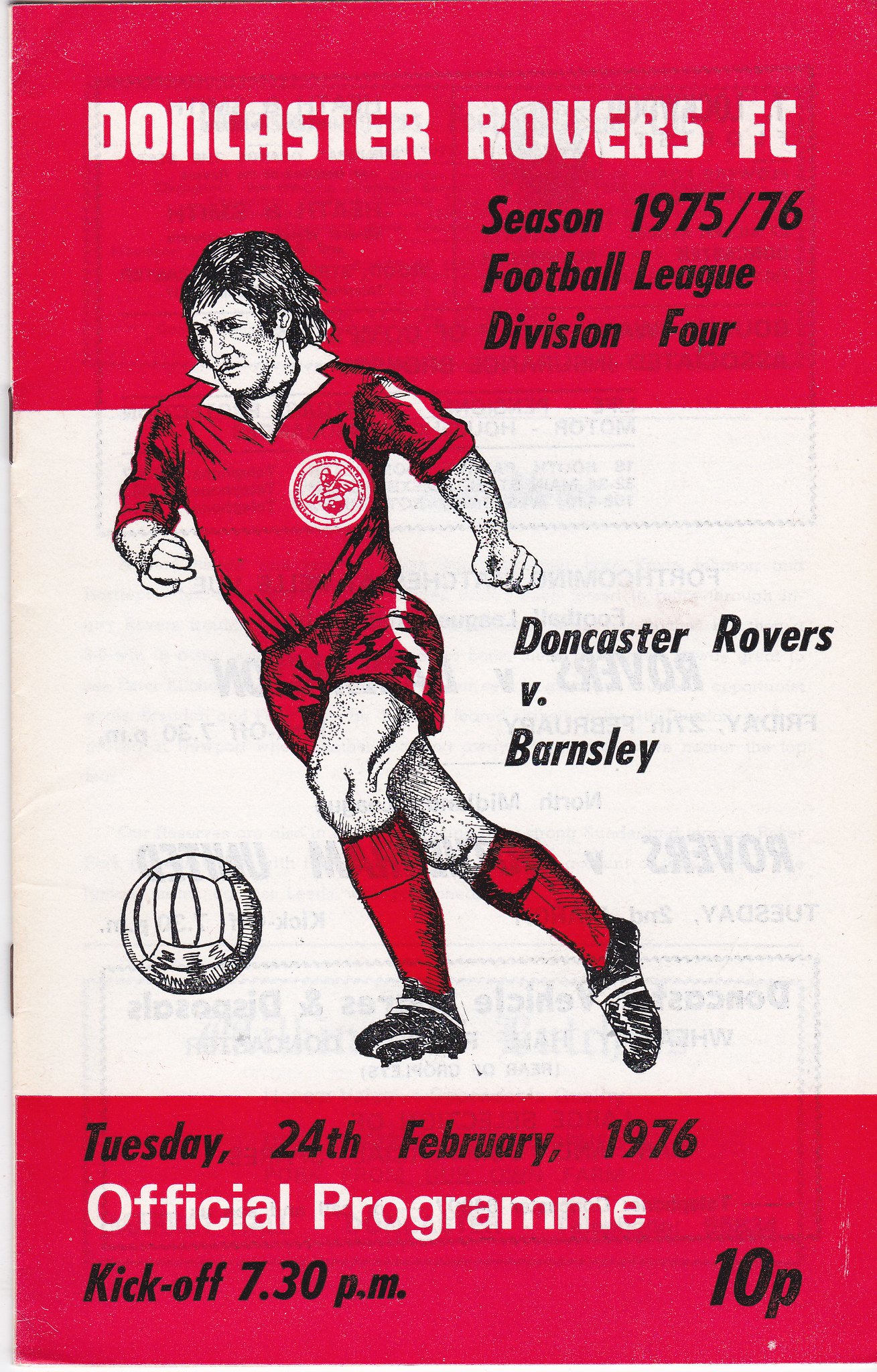A detailed poster for a football league match features prominently at the top, a red bar with "Doncaster Rovers FC" in white text. Right below, in black text, it states, "Season 1975-76 Football League Division 4." Beneath this text, there is a semi-realistic animated image of a footballer in mid-action, dressed in a red jersey with a white collar and white stripes running down the arms and shorts, paired with red socks just below the knee. The footballer, with medium-length hair, is depicted just about to kick a ball. To his right, in black writing on a white background, it reads, "Doncaster Rovers V Barnsley." Further down is another red strip, with black text indicating, "Tuesday 24th February 1976." Below this, it states, "Official Programme" (using the archaic "e" spelling) and "Kick-Off 7.30 p.m." On the far right, the price is listed as "10p." The overall layout clearly advertises the football match details, emphasizing the team, date, kickoff time, and admission cost.